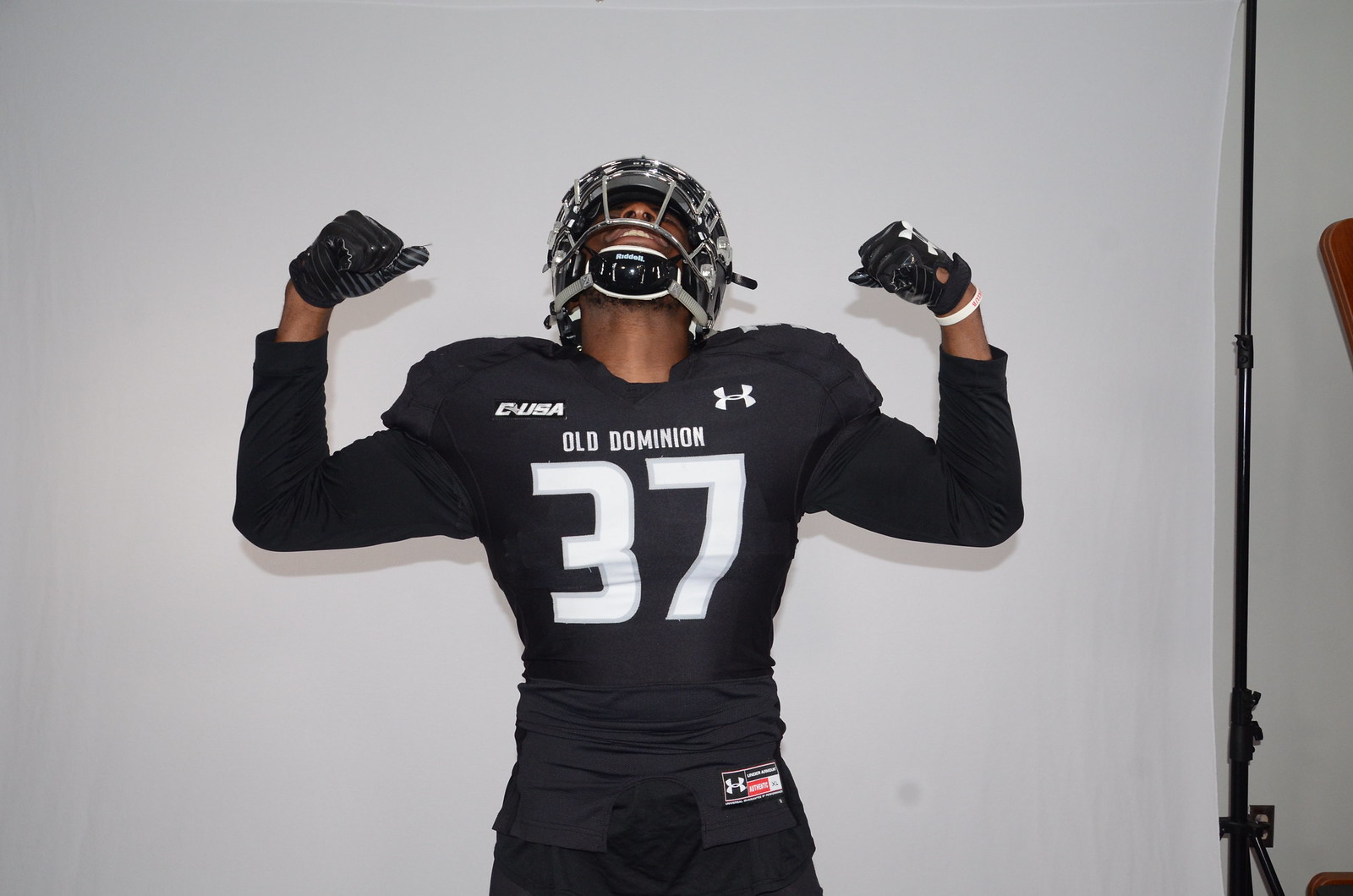In this detailed image, an African American male is prominently displayed against a white background, which could be a screen or wall, with some brown elements and a stand visible to the right. The individual is dressed as an American football player, clad in a black jersey adorned with several white logos and inscriptions. At the top left of the jersey, the white letters "CUSA" are clearly visible, while the top right features the Under Armour logo in white. Centered on the chest, the jersey proudly displays "Old Dominion" and the large white number 37. Beneath these, there are additional smaller logos, one of which appears to be an 'H' in a spiral design.

The player is equipped with a black helmet, which has silver detailing. His jersey, supplemented with padded shoulder armor, has long black sleeves. He is also wearing black gloves with white detailing on the top and a white rubber bracelet on his left wrist. 

The athlete’s stance is striking; he is looking upwards with his head tilted back, eyes closed, mouth open as if shouting towards the sky. His arms are raised and bent at the elbows, fists clenched tightly as if in the midst of an intense celebration or exertion, giving the impression of a powerful, victorious or emotional moment. His entire appearance, amidst the clean and stark backdrop, emphasizes his dynamic energy and the detailed intricacies of his uniform and gear.